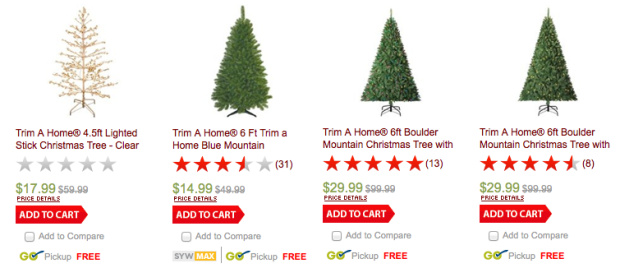This image showcases a detailed storefront page from a retail website, specifically featuring a selection of Christmas trees. The background of the page is a clean, white backdrop, highlighting four distinct Christmas tree listings.

1. **First Tree**: The brand is Trim A Home, featuring a 4.5-foot lighted stick Christmas tree. The tree is minimalistic, essentially a bare stick adorned with lights. It is currently on sale for $18, discounted from $60. This tree has no customer ratings yet.
   
2. **Second Tree**: A Home Blue Mountain Tree, priced at $15. This tree has received a 3.5 out of 5 stars rating, based on 31 customer reviews.

3. **Third Tree**: The Boulder Mountain Christmas Tree, priced at $30. It boasts a perfect 5 out of 5 stars rating, derived from 13 customer reviews.

4. **Fourth Tree**: Another Boulder Mountain Christmas Tree, this one is 6 feet tall and also priced at $30. It holds a 4.5 out of 5 stars rating, with 8 customer reviews.

Underneath each tree listing, there is an option to add the item to the cart, and all items are available for pickup as well as free shipping.